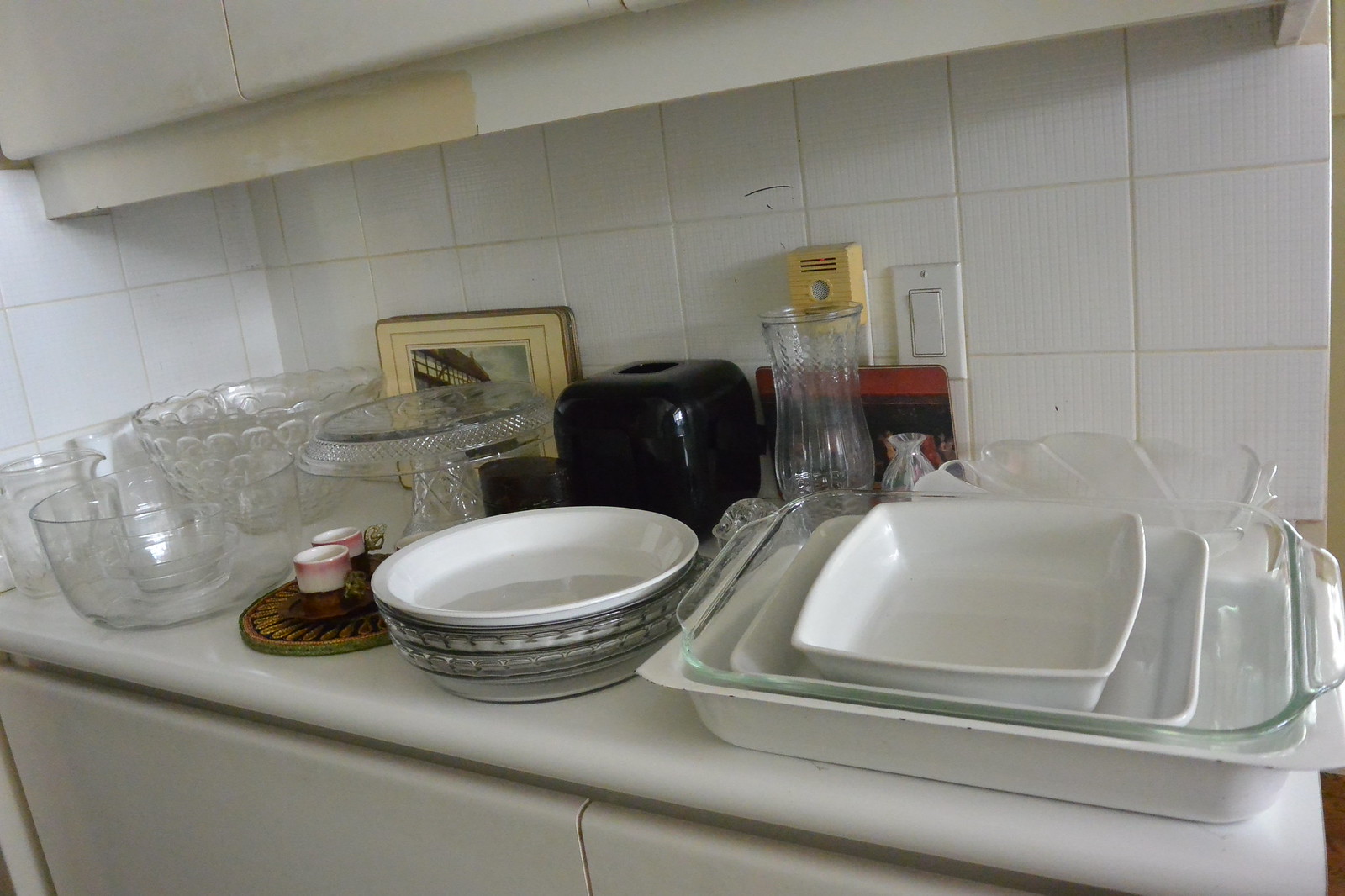A charming photograph of a vintage kitchen counter showcases an eclectic collection of antique dishware. On the right side, a stack of square glass dishes of various sizes is seen, topped with a white dish holding a translucent glass dish, which in turn contains two smaller white ceramic dishes, all neatly nested together. To the left, a bowl featuring a striking gray and black design with a white interior adds a touch of artistry. Behind this bowl, a black bread box and a flower vase are visible, accompanied by a wall-mounted yellow box and a light switch adjacent to it. Further to the left, a crystal cake stand with an intricate design draws attention. In front of this stand, a small wooden plate holds two delicate white cups adorned with a pink outline around their lips. Contributing to the vintage ambiance, additional glass bowls are placed on the far left. The setting evokes nostalgia, reminiscent of a cozy kitchen from a grandparent’s home, filled with cherished, timeworn treasures.